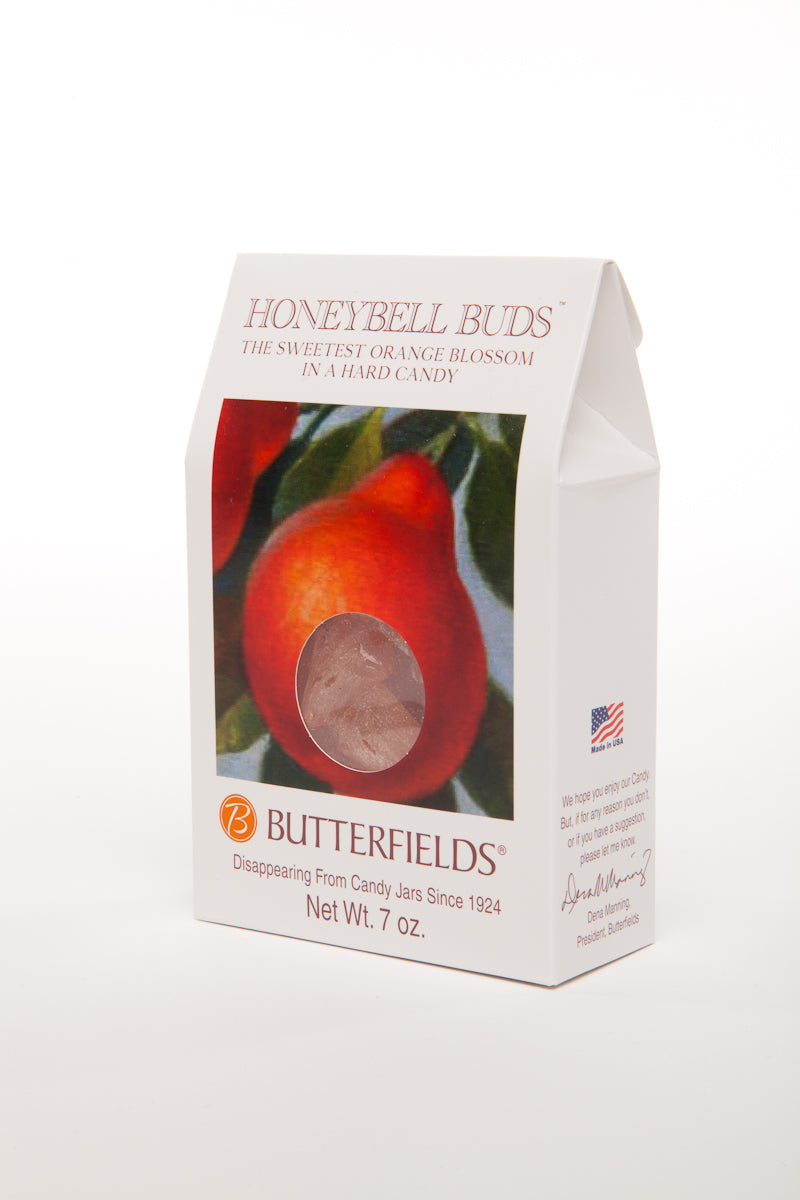The photograph showcases a white bag of hard candy titled "Honey Bell Buds," described as the sweetest orange blossom in a hard candy. The center of the package features red-orange text that reads "Honey Bell Buds," with a photograph of a pear-shaped orange situated beneath it. The packaging includes a plastic window, offering a glimpse of a couple of the long, brown candies inside. At the bottom, the text reads "Butterfields, disappearing from candy jars since 1924," with an adjacent image of a bee inside an orange circle, likely the company's logo. The package also specifies a net weight of 7 ounces. Alongside, there's an American flag with the statement "Made in USA" beneath it. Following this is a note from the company president, Dina Manning, that says, "We hope you enjoy our candy, but if for any reason you don't, or if you have a suggestion, please let me know," with her signature below. The bag is positioned in the center against a white background and surface, slightly angled to the left, creating a clean and uncluttered presentation.